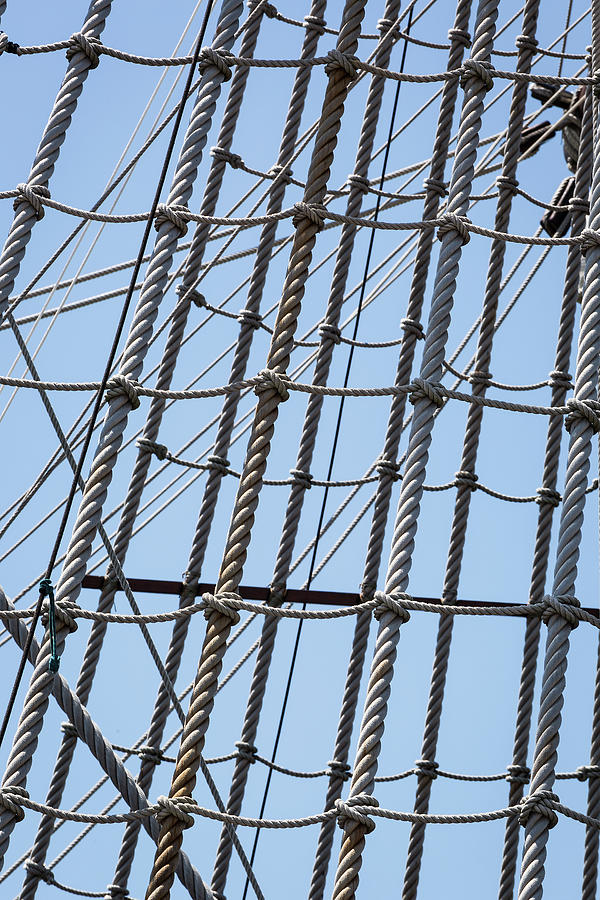The photograph captures a close-up view of the intricate rigging on a sailing ship, set against a clear, cloudless light blue sky typical of a bright daytime scene. The composition is rectangular, with its longer sides aligned horizontally. Central to the image is a dense, net-like pattern formed by intertwining large, thick ropes of varying hues such as white, tan, and brown. These ropes are meticulously bound together by thinner strands, creating an organized, layered look. At an angle, running diagonally from the bottom left to the top right of the frame, several single thin strands of rope lead towards what appears to be a slightly off-screen ship's mast. In the top right corner, the presence of multiple pulleys adds to the scene's complexity. The comprehensive layering of ropes, along with their intersecting patterns, evokes the essential structural elements of a sailing vessel's rigging system.